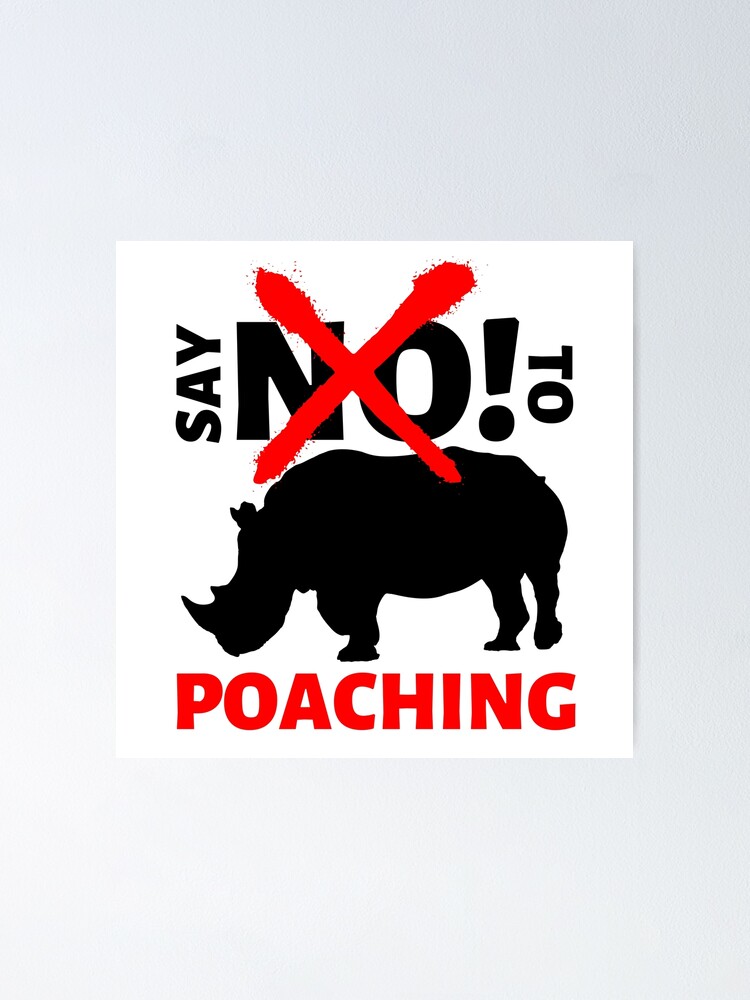The illustrated sign, set against a blue background with a central white square, emphatically declares "SAY NO TO POACHING!" The black silhouette of a rhinoceros with its head lowered and a large horn dominates the center. The bold word "NO," capped by an exclamation point, is strikingly overlaid with a large red X, part of which intersects the rhino's back. Flanking the rhino, the words "SAY" and "TO" are oriented vertically on either side of "NO," while "POACHING" is printed in vivid red capital letters at the bottom. This powerful visual message urges viewers to reject poaching.